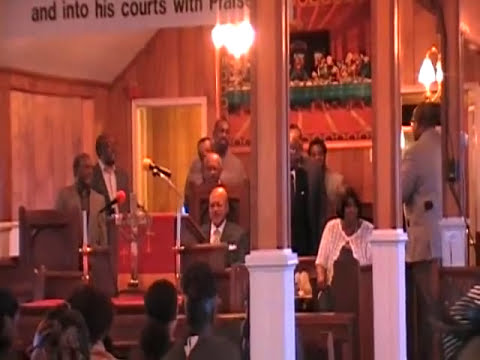The image depicts the interior of a church during what seems to be a religious ceremony or worship service. The scene is viewed from the perspective of the pews, where several people are seated, dressed in dark clothing. Up front, there are multiple podiums equipped with microphones, surrounded by individuals standing or sitting in chairs. Behind them, a large depiction of The Last Supper adorns a wooden wall. The architectural details include white beams extending up to the ceiling, transitioning into wooden columns. Partially visible at the top left of the image is a banner with black text on a white background that reads "and into his courts with." There is no indication of musical instruments, suggesting the focus may be on vocal performances. An open door is visible behind the people at the podiums, highlighting the depth of the space.